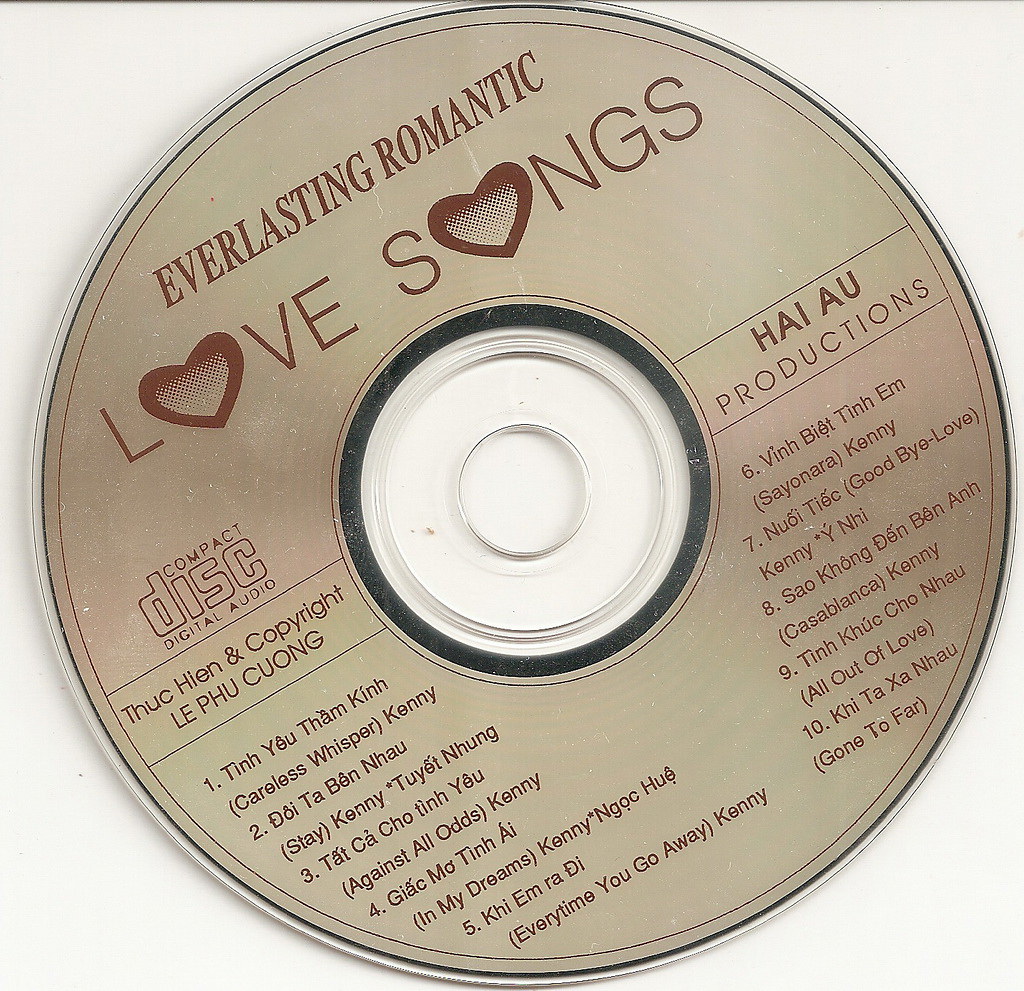The image showcases a single, centrally-placed CD against a white background. The CD features a silver label adorned with various colors including white, silver, maroon, and black. Prominently, in maroon at the top, it reads "Everlasting Romantic Love Songs," with the O's in "Love" and "Songs" stylized as hearts. Below this title, the CD displays additional text, likely in Thai, and an inscription that includes "Compact Disc Digital Audio," "Thookian," and "Copyright." The label is divided into two segments; the left side lists songs 1-5 and the right side lists songs 6-10. These song titles include both the original foreign language and their English translations, such as "Careless Whisper," "Stay," "Against All Odds," "In My Dreams," "Every Time You Go Away," "Sayonara Goodbye Love," "Casablanca," "All Out Of Love," and "Gone Too Far." The bottom half of the label features "H-A-I-A-U Productions" written at an angle. The overall layout emphasizes both the aesthetic and informational elements of the CD, positioning it as a collection of classic romantic tracks.